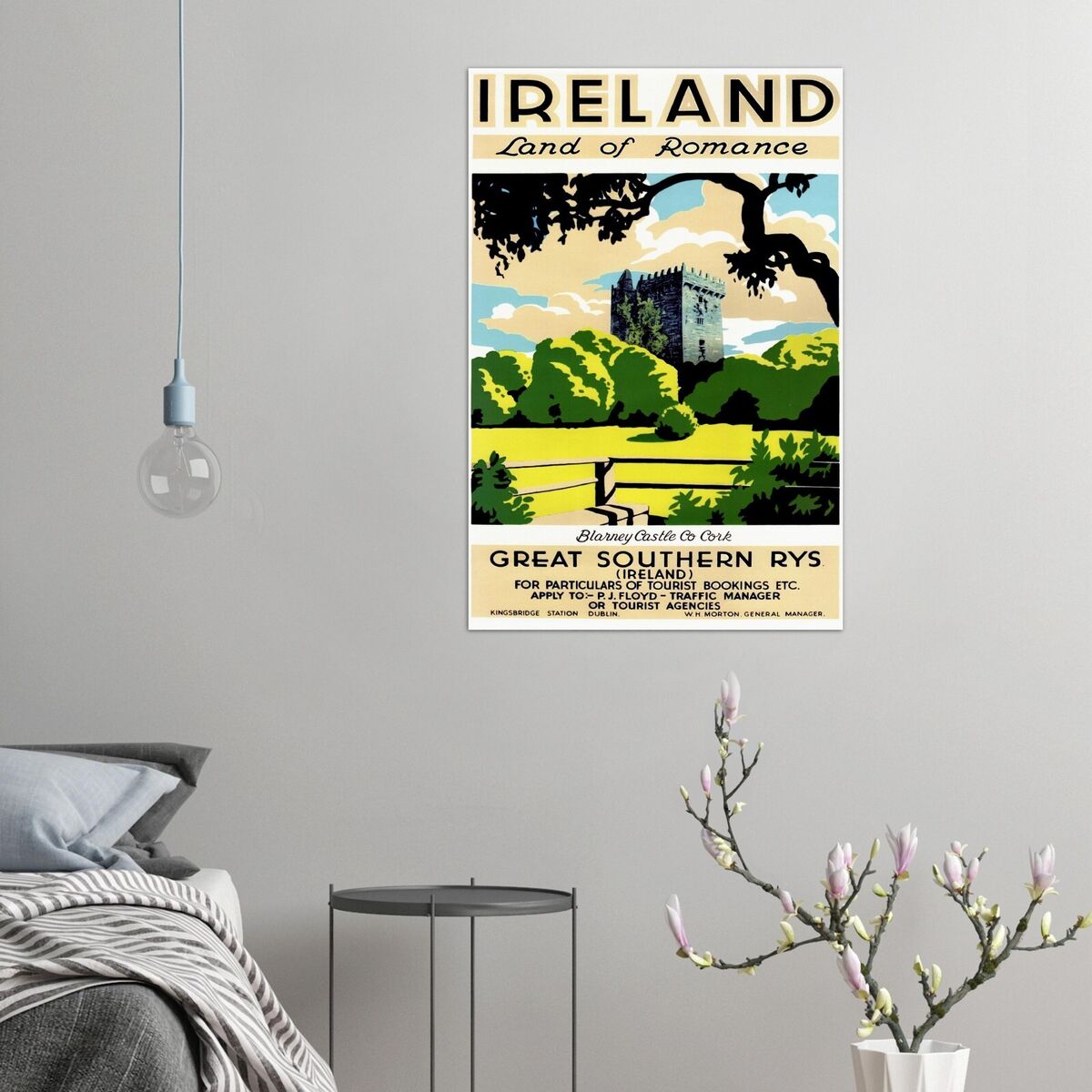The photograph showcases a cozy bedroom with off-white walls. In the lower left corner, there's an unmade bed with partially pulled-back, gray and white striped covers, and a mix of gray and darker gray pillows, including one light blue pillow. Adjacent to the bed, a small, dark gray, round metal bedside table holds a minimalist white vase containing thin twigs with light pink, unopened blossoms. Near the bed hangs a lightbulb on a lengthy, baby blue cord from the ceiling. The upper left part of the image features a poster with a blend of white, tan, green, brown, and a touch of blue colors, prominently displaying the title "Ireland, Land of Romance" in black letters. The poster depicts a scenic view from a small balcony with a railing, looking towards a castle surrounded by large shrubs and trees, and includes details such as "Barney Castle, Cork, Great Southern RYS, Ireland" and tourist information directed to PJ Floyd, Traffic Manager, King Sirk Station, Dublin.